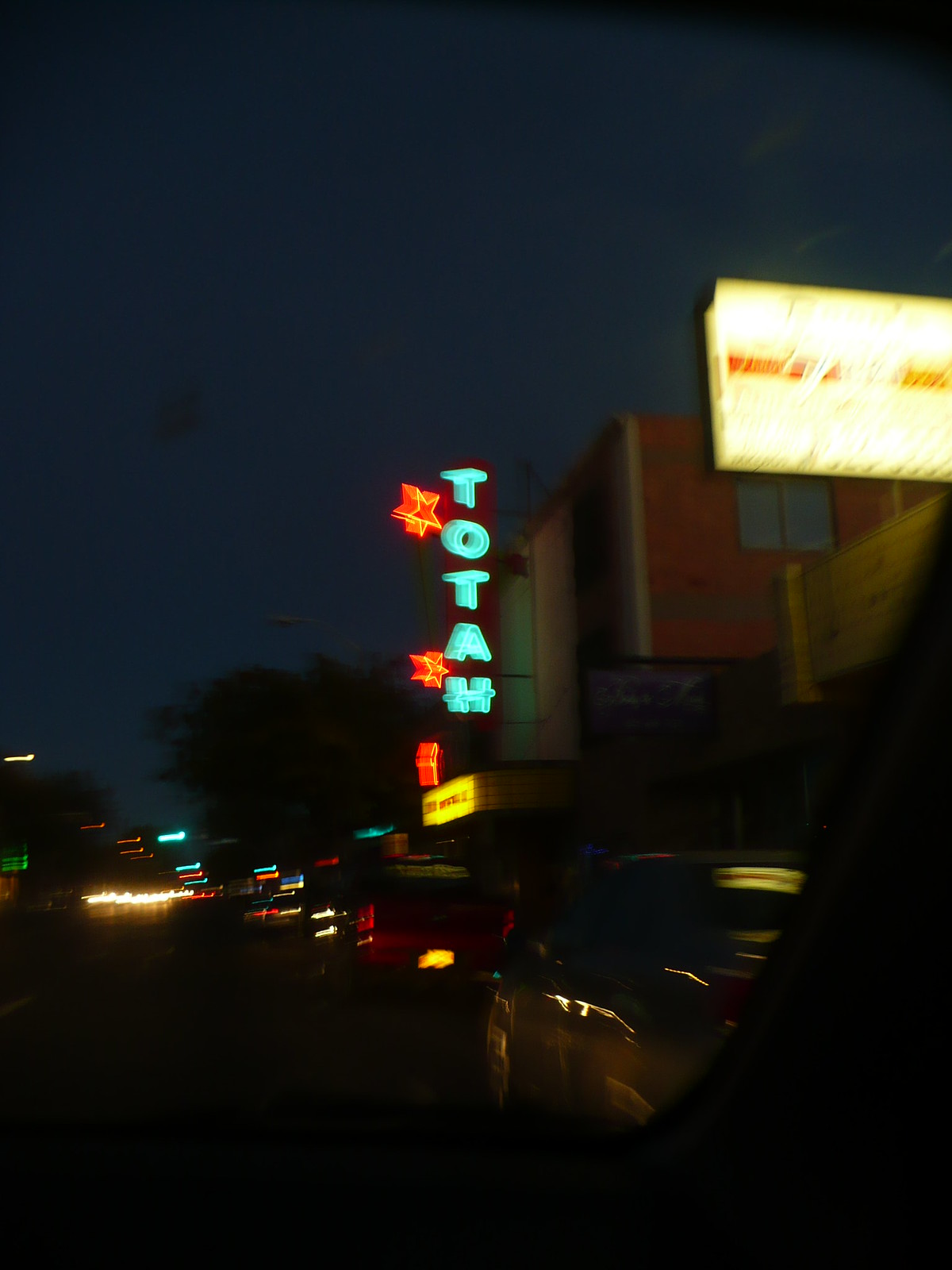This is a blurry nighttime image of a commercial street scene. Multiple brightly lit signs adorn the fronts and sides of buildings, one with a yellow background and red lettering, though the text is illegible due to the blur. Another prominent sign is vertical, reading "TOTA," with the letters in blue and accompanied by three red stars. The dark sky is dimly lit by streetlights and numerous car headlights, some of which appear stretched and distorted due to the camera shake. Parked cars, possibly black or silver, line the street, contributing to the busy, albeit unclear, nocturnal setting. Overall, the image fails to capture anything in sharp focus, making details difficult to discern.